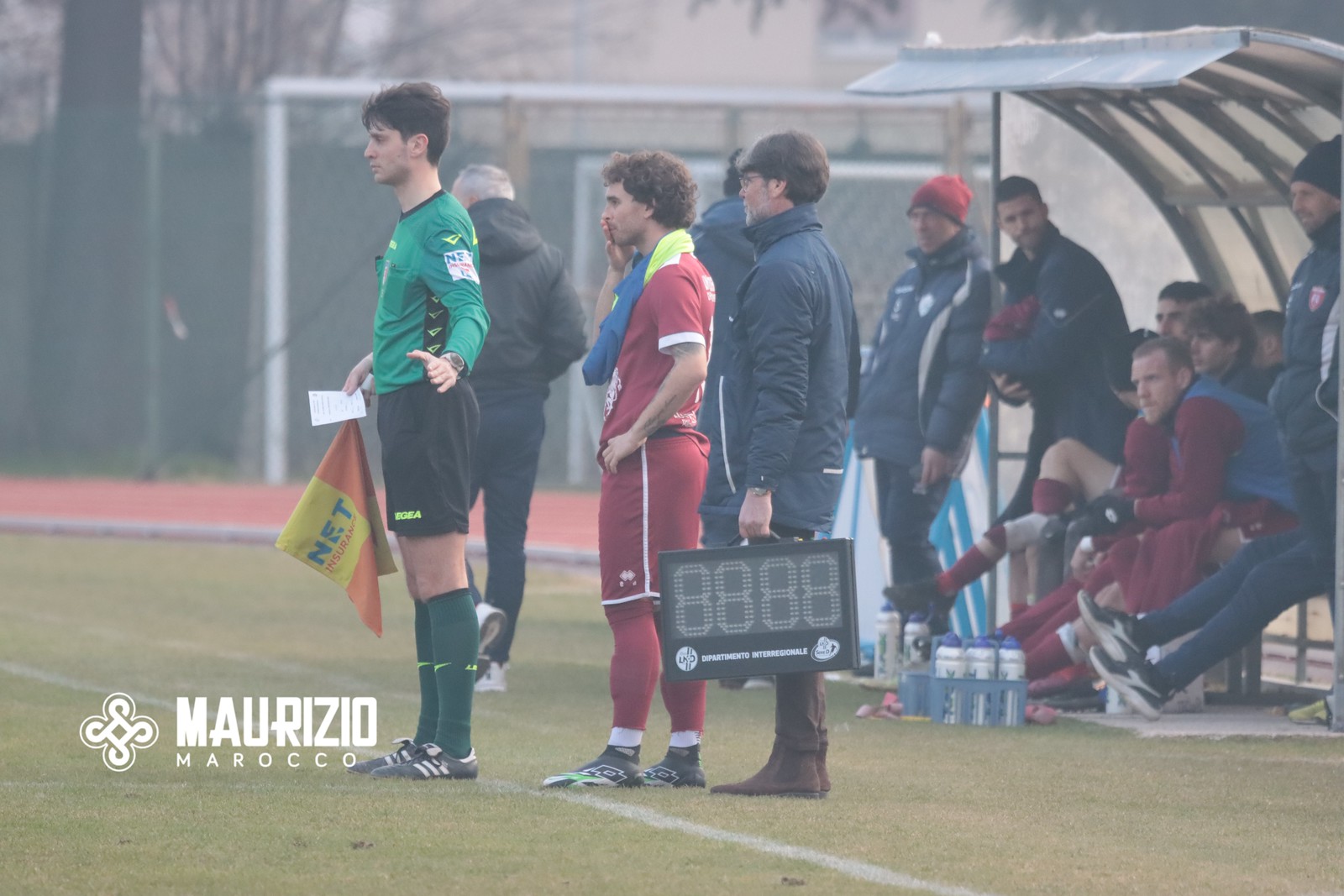The photograph captures an outdoor soccer game on a cold, foggy day, evidenced by the players and staff wearing heavy jackets and down vests. The scene shows the sideline, where several individuals are gathered, some seated under a half-moon-shaped shelter for warmth. Prominently featured is a young, tall sideline judge dressed in a green long-sleeve shirt, black shorts, and knee-high forest green socks. He holds an orange and yellow flag in his right hand and wears black cleats. To his left is the timekeeper with the score box, not turned on, and there's a water bottle carrier nearby.

In the background, players in maroon-red uniforms with white accents are visible, along with additional soccer goals and distant trees, indicating an urban setting with large buildings. A man in a red jersey, red shorts with white accents, and deep red leggings stands slightly behind the sideline judge. At the bottom left corner of the image, the text "Maurizio, Morocco" suggests the location being Morocco. The overall atmosphere hints at chilly conditions without precipitation, amidst the visible faint fog and the diverse assembly of players, coaching staff, and officials on the soccer field.